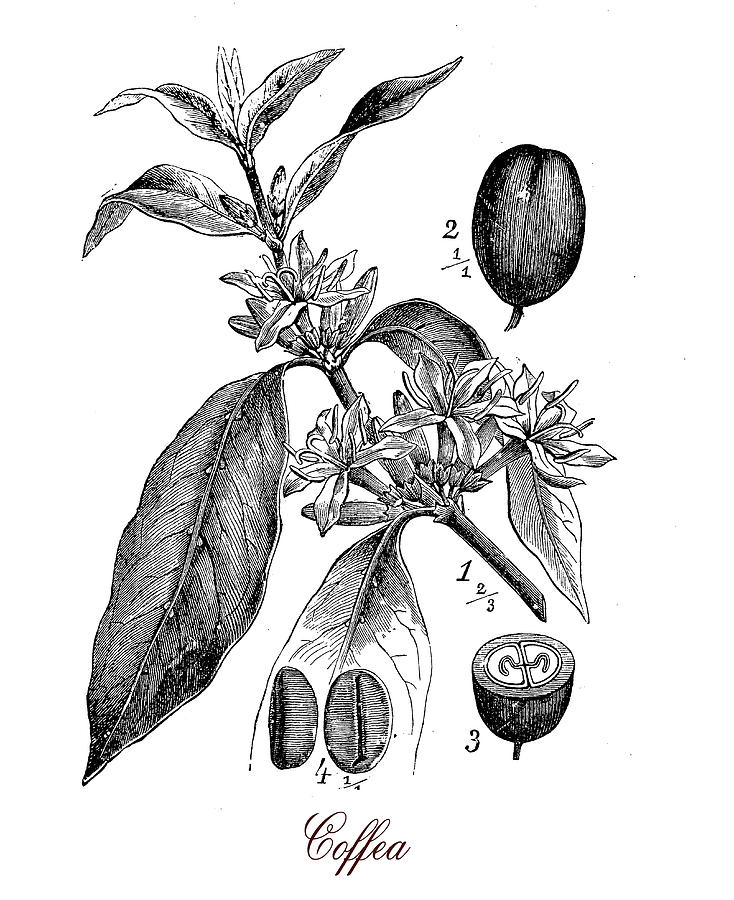The image is a black and white pen and ink botanical illustration of a coffee plant, meticulously detailed with fine lines. The plant is identified as a coffee plant through the word "coffea" written in an elegant, brown calligraphy at the bottom of the sketch. The illustration features the flowering tip of a coffee bush branch, showcasing smaller leaves at the tip and progressively larger leaves down the stem. Several whorls of coffee flowers are visible at different leaf nodes along the stem. Additionally, the sketch includes various measurements scattered throughout, such as "2 and 1 out of 1," "1 and 2 thirds," "3," and "4 and a quarter," though their exact references remain unclear. Off to the side, separate drawings illustrate different stages of the coffee fruit and beans: one shows the whole fruit, another depicts the fruit cut open to reveal the beans inside, and a third drawing focuses on two halves of a coffee bean superimposed on the bottom leaf, emphasizing the intricate structure normally seen in whole coffee beans. The entire illustration is rendered against a white background, highlighting its detailed, historical aesthetic.